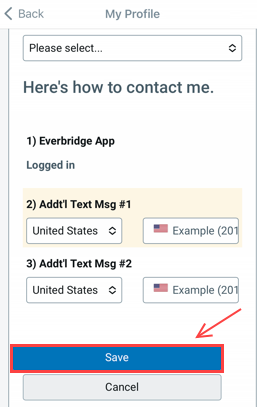The image is a screenshot of a messaging platform interface. At the very top center, the phrase "My Profile" is displayed in a light gray color. On the top left, the word "Back" accompanied by a left arrow is also shown in the same light gray color. Below this header, there is a rectangular box featuring the text "Please select..." on the left side in black font, while the right side of the box contains an up and down arrow intertwined.

Further down, text reads, "Here’s how to contact me." This is followed by a list numbered one to three. Next to number one, the name "EverBridge App" is displayed in black text with the status "Logged in" below it. Position two reads "Add additional text message number one," with a rectangular box underneath containing the text "United States" on the left and another box on the right displaying an American flag icon and the word "example." Similarly, position three says "Additional text message number two," accompanied by the same "United States" text and flag icon arrangement.

At the very bottom of the image are two prominent rectangular buttons: the top button labeled "Save" and the bottom button labeled "Cancel."